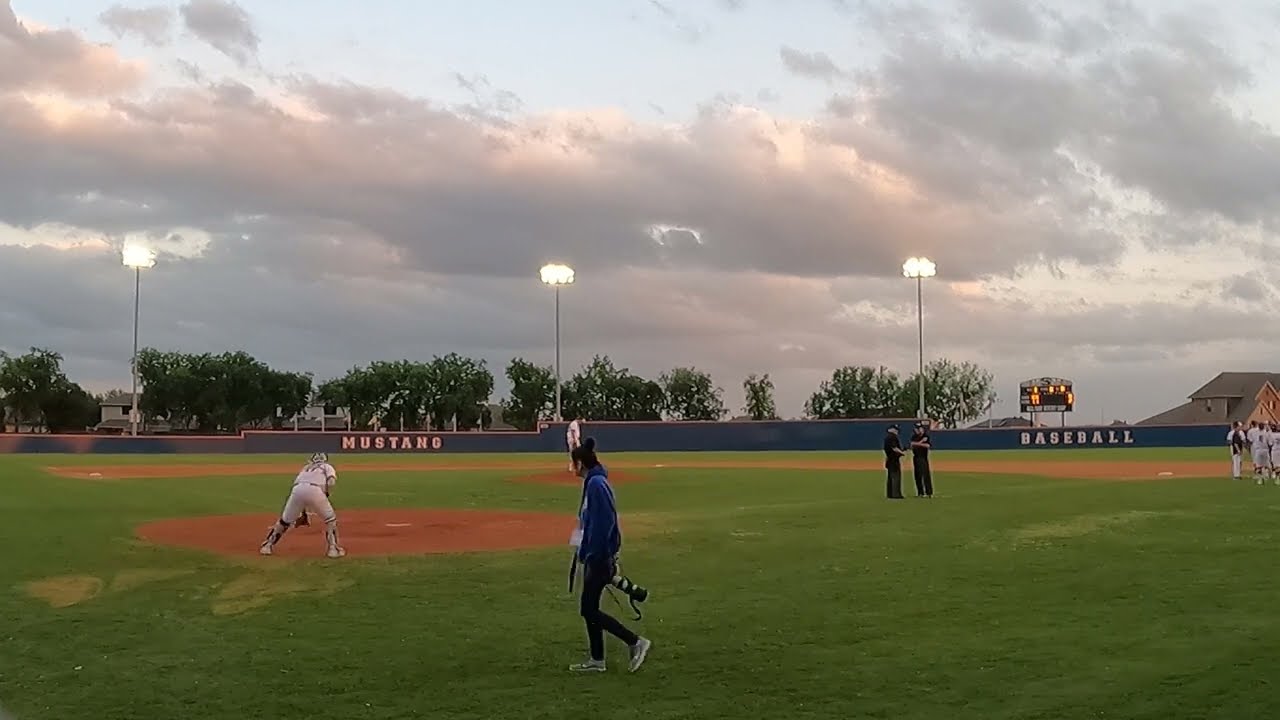This image captures a dynamic moment on a baseball field, viewed from behind home plate. Centered prominently is the catcher, outfitted in white and blue gear, indicative of his role. In the foreground, a photographer with dark hair, wearing a large purple shirt or possibly a blue hoodie and black jeans, walks through the scene holding an imposing camera with a long lens. Just left of center, two umpires dressed in black converse, while off to the right near the edge of the frame, four or five players engage in discussion near first base. Stretching across the background, three tall overhead lights illuminate the field, casting their glow over the green grass and dirt areas, including around home plate and the pitcher's mound where a pitcher in white stands. The back wall of the field prominently displays the words "Mustang" and "Baseball," next to a partly legible scoreboard. Surrounding the field, six or seven trees stand under a partly cloudy sky. The main colors throughout the scene include green, white, gray, and blue. The overall atmosphere suggests a lull in the game action.